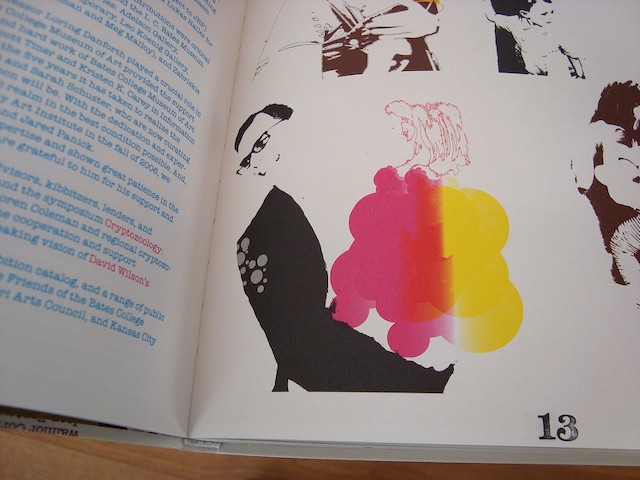The image shows the inside of an open book, specifically page 13 on the right side of the binding. This right-hand page features multiple art illustrations and sketches. Dominant among these is a faint black-and-white sketch of a man with short hair and glasses, juxtaposed next to a vivid red, orange, and yellow smudge that seems to represent a woman with her dress. Above this, there's a small black-and-white sketch of a baby. To the left of the baby, there is another sketch, though the details of this are unclear. 

Further to the left, partially obscured, is another figure that appears seated mid-page. In addition, silhouettes of people's heads and hands seem to fill the page, but these remain somewhat indistinct. 

On the left-hand page, which is harder to read due to the angle and small text, there are words like "cryptozoology" and "David Wilson" visible amongst the text. This left page seems to contain a detailed blueprint or textual content relevant to the images.